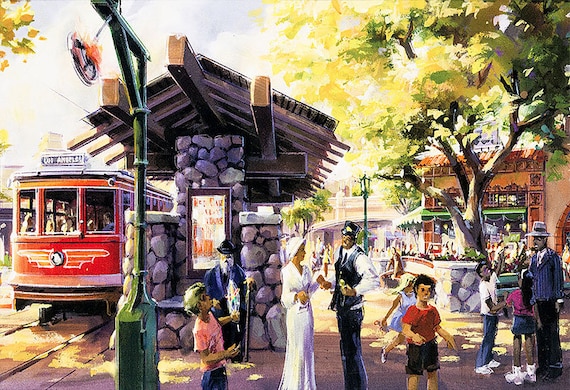This vibrant painting, likely an acrylic piece, captures a bustling scene from what appears to be a mid-20th century town square, reminiscent of places like San Francisco. The left side prominently features a bright red streetcar, adorned with white accents and some illegible text at the top, moving along tracks that curve towards the viewer. The streetcar is populated with people, giving it a lively feel.

Adjacent to the streetcar is a stone-built pavilion, serving as a trolley stop. This structure boasts a sturdy stone foundation made of round rocks, with matching pillars supporting a roof accented by wooden details. A green lantern hangs in front of the pavilion, adding to its quaint charm. A sign, likely indicating the streetcar's route, is mounted on one of the stone pillars.

Across the scene, there are various figures engaged in conversation and activity. A woman in white converses with what appears to be a trolley conductor, and other individuals, dressed in period attire such as suits and hats, indicative of the 1940s, are scattered around. Notable is a man in a blue suit, a person in pink, and another in red.

The backdrop is filled with a mix of shops and buildings, hinting at the painting's depiction of a lively public plaza. Dominating the scene is a large oak tree, its gold-hued leaves suggesting a fall setting, planted in a square stone planter. The sunlight filters through the clouds, casting warm light across the scene but also creating shadows where people seek respite.

Period light posts, which look like the kind manually lit in older times, dot the square, enhancing the nostalgic ambiance. The overall bright, day-glow color palette of the painting, coupled with the detailed depiction of everyday life, captures a picturesque moment, reflective of a peaceful, bygone era.